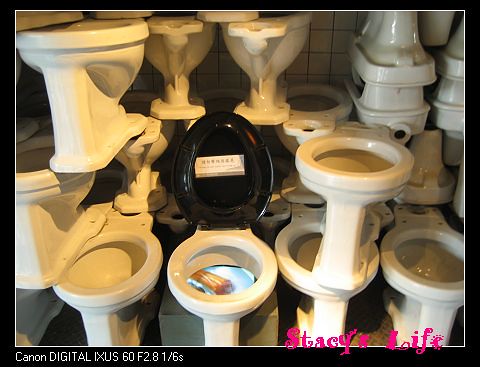The image depicts an arrangement of twelve white porcelain toilets stacked against a white tiled wall with dark grout lines, possibly in a shop or a recycling facility. The tiles are relatively small, possibly 6 or 9 inches in size. The toilets are organized in three rows: four on the bottom, four on a middle tier, and four more on the top tier. All except one in the center lack any hardware or back tanks. The central toilet, distinct with a shiny black seat and lid, has its seat lifted. Inside its bowl is an illuminated green light and a light beige mass. On the underside of this toilet’s lid is a label with what appears to be Japanese or Chinese characters. In the bottom left corner of the image, white text on a black border reads "Canon Digital iXUS 60F2.8 1/6S." In the bottom right corner, pink text reads "Stacy's Life."